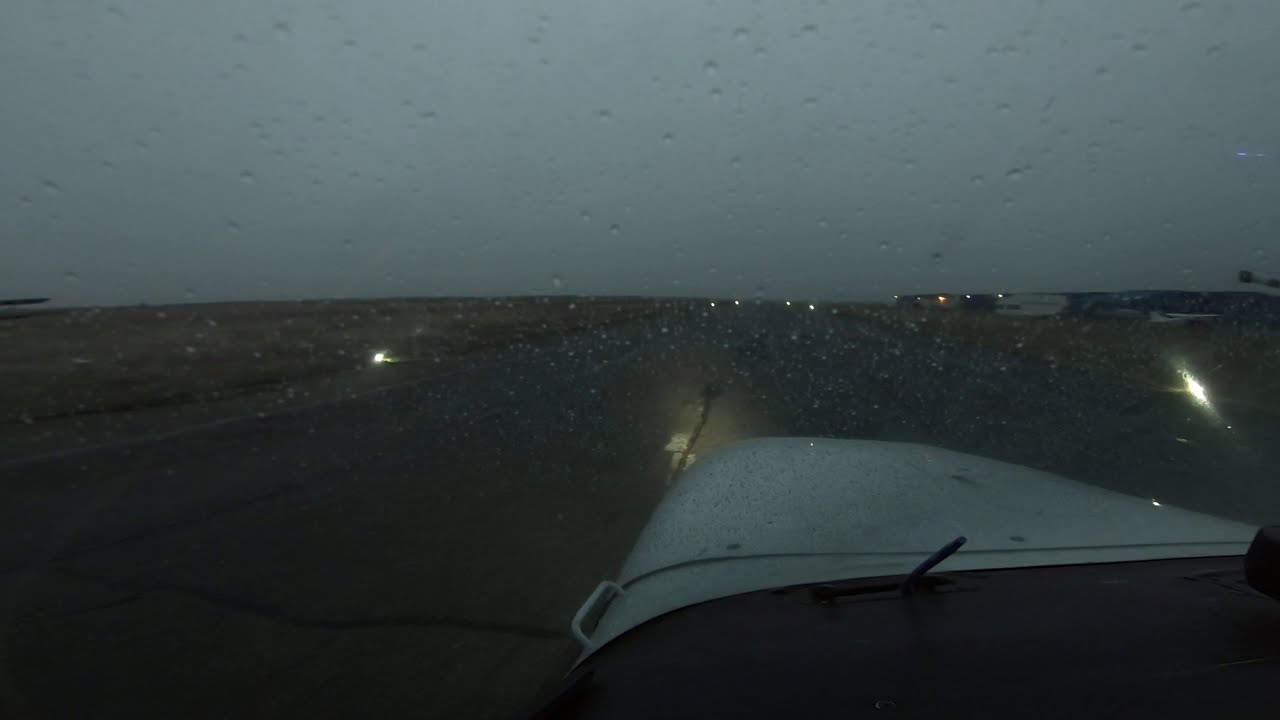The image captures a dusk or early morning scene from the vantage point of looking out of a windshield, likely that of a plane or car. The scene is dimly lit under an overcast sky, which casts a grayish hue over the entire landscape. Raindrops are scattered across the windshield, hinting at a recent or ongoing drizzle. Ahead, a road or runway stretches into the horizon, bordered by fields of brown grass. To the right, distant vehicles and a large, gray, warehouse-like building are visible. The vehicle's hood, possibly white, and a flattened dashboard are in the foreground. Off in the distance, glowing lights illuminate parts of the landscape, including a low structure in the center of the frame, suggesting an airport environment. Choppy waters or a seashore on the left adds a dynamic element, though partially obscured by the low light. Red and white colors on a wing tip, visible through the raindrops, further confirm the airplane vantage point. Various lights marking the runway guide the eye to a vanishing point where the runway disappears into the horizon.